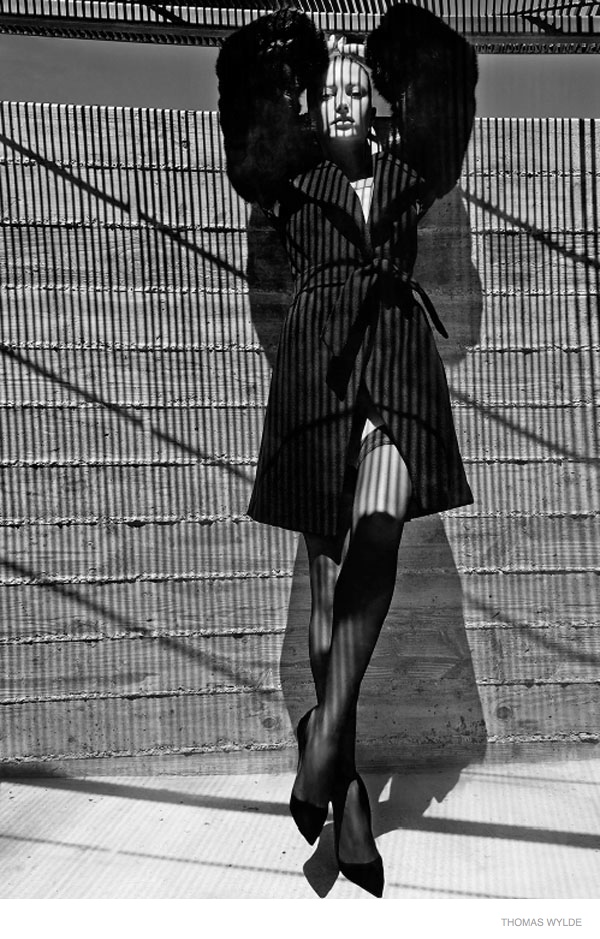In this striking black-and-white fashion photograph, a tall young woman stands poised against a textured concrete wall, exuding elegance and sophistication. She is draped in a luxurious black wrap coat by designer Thomas Wilde, which features dramatic puffy sleeves and is cinched at the waist with a belt. The coat casts intriguing shadows under a grate, creating a captivating pattern of vertical and diagonal lines that play across her figure and face.

Her posture is confident, with her right leg crossed over her left, and her arms gracefully clasped behind her head. Though it is challenging to discern the exact length of her hair, it appears to be styled up, possibly in a bun, suggesting an air of refined simplicity. She wears black high-heeled pumps and nylon stockings that ascend to her thighs, completing her chic ensemble.

The high contrast in the image highlights both intense darks and luminous whites, enhancing the dramatic effect of the lighting and shadows. The setting appears to be outdoors, with the woman standing on concrete, adding a raw, urban edge to the overall aesthetic. The photograph's textural background and the complex interplay of light and shadows make it a visually arresting piece, capturing the essence of high fashion in a moment of still elegance.